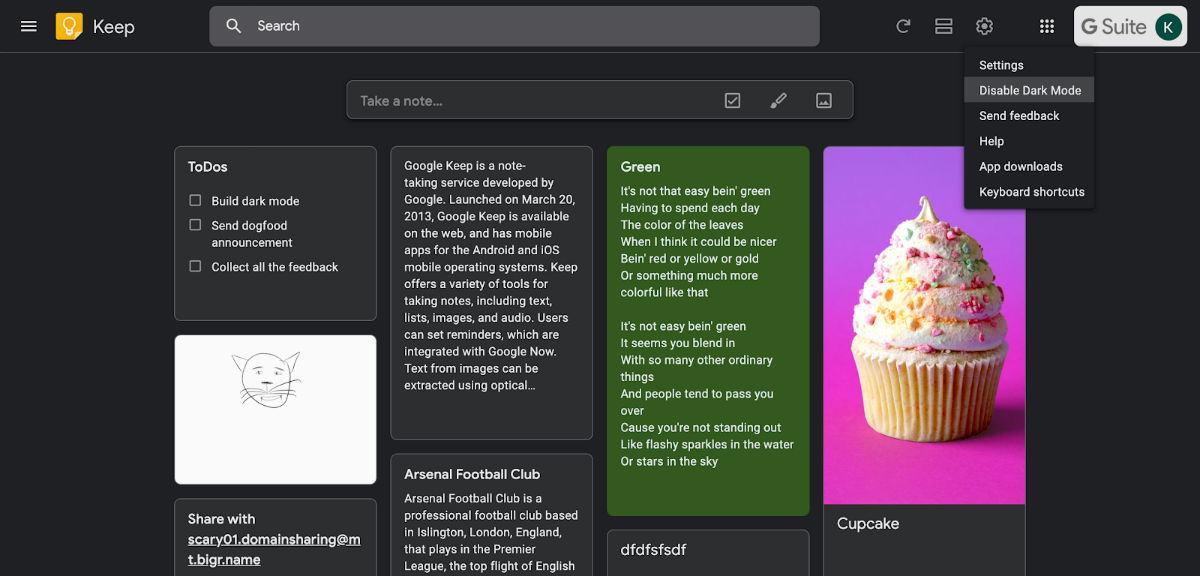### Detailed Caption for Website Screenshot

The image is a screenshot of a website featuring a predominantly black background. At the top left, there are three horizontally-stacked white lines commonly known as a "hamburger menu." Adjacent to this icon is a light orange square with a white border and a light bulb symbol in the center. Next to the icon is the word "Keep" written with a capital 'K'.

Moving rightward, there is a light gray search bar with a white magnifying glass icon and the word "Search" also beginning with a capital 'S'. Outside of the search bar, the background remains black featuring a refresh icon depicted by a white arrow. Following this is an icon of two stackable rectangles and a sprocket, indicating the settings menu. The sprocket icon appears clicked, revealing a dropdown menu with options such as "Settings," "Disable dark mode" highlighted, "Send feedback," "Help," "App downloads," and "Keyboard shortcuts."

Above this menu, there is a square grid with nine white dots next to a rectangular box with rounded edges containing a large gray letter 'G' on a white background, followed by 'Suite' with a capital 'S' and a dark green circle housing a white letter 'K.'

Below this is another search area bordered in gray with the placeholder text "Take a note" in light gray. To the right are a series of action icons: a white-bordered box with a white checkmark, a pencil icon with a white tip, and another icon representing mountains within a box. 

The lower section displays four vertical boxes. The first box, labeled "Todos" in one word with a capital 'T' and 'D,' contains three sub-boxes with the tasks: "Build dark mode," "Send dog food announcement," and "Collect all the feedback."

Beneath these tasks is a small square displaying a child's drawing of a cat, featuring whiskers, ears, round face, and human-like eyes. Below this image, a box with a gray border contains the word "Share" with a capital 'S'. Following this is a text box that reads "the website of scary01.dom, domain sharing at mt.bigr.name."

Adjacent to this, a black background box with white text explains, "Google Keep is a notes taking service developed by Google. Launched on March 20th, 2013. Google Keep is available on the web and has mobile apps for Android and iOS. Keep offers a variety of tools for taking notes, including text, lists, images, and audio. Users can set reminders, which are integrated with Google Now. Text from images can be extracted using optical..." and cuts off.

Followed is another gray-bordered box with "Arsenal Football Club" mentioning the club is based in Islington, London, and plays in the Premier League. The text cuts off after "the top flight of English."

The next box is rectangular with a dark green background and the word "Green" in capital letters at the top. The text within reads: "It's not that easy being green, having to spend each day. The color of the leaves, what I think it could be nicer being red or yellow or gold or something much more colorful like that."

Further down, a paragraph continues with: "It's not easy being green. It seems you blend in with so many other ordinary things. People tend to pass you over because you're not flashy like sparkles in the water or stars in the sky."

At the bottom of the screenshot, a partially visible gray-bordered area contains the lowercase string "dfdfsf sdf sdf." To the right, a rectangular pink background showcases a cupcake with white frosting, sprinkled with pink, blue, and yellow decorations. The cupcake base has a yellow ridged liner, and below this image, the word "Cupcake" is written with a capital 'C'.